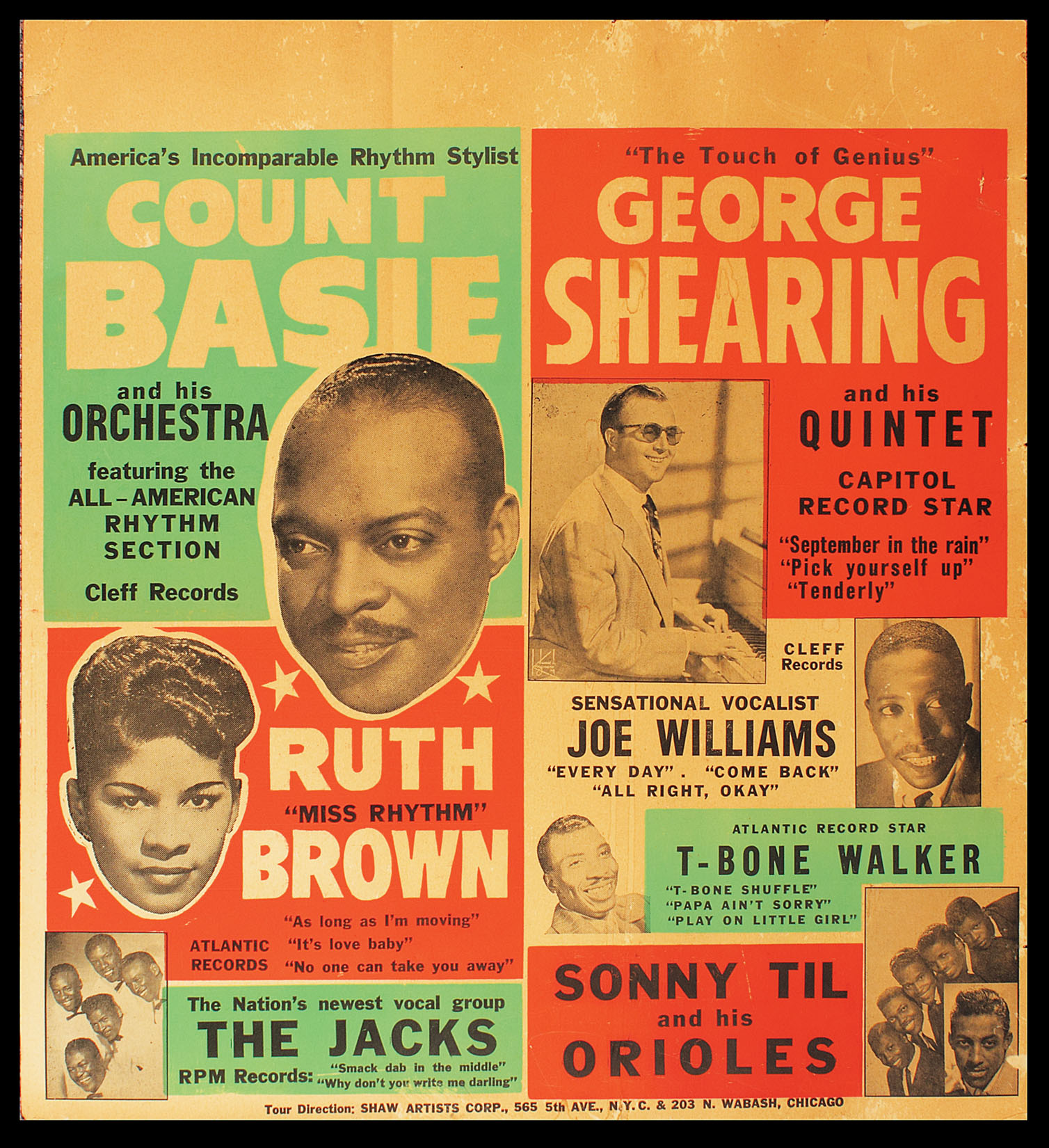This image is a detailed poster or magazine clipping, likely from the 1950s or 1960s, showcasing various prominent musicians and vocal groups. At the top, the text reads "America's Incomparable Rhythm Stylist" and "The Touch of Genius," highlighting Count Basie and his orchestra, featuring the all-American rhythm section on Clef Records. Adjacent to this, "George Shearing and his quintet, Capitol Record Star" is prominently mentioned, with some featured songs including "September in the Rain," "Pick Yourself Up," and "Tenderly."

In the center of the poster, "Ruth Brown" is displayed in bold white text on a red background, with "Miss Rhythm" elegantly written in black text across her name. The poster also promotes the nation's newest vocal group, "The Jacks" listed as being with RPM Records, and features an image of five African-American men in the bottom left corner. Near the bottom right corner, there's another group of African-American men highlighted, which includes "Sonny Till and his Orioles." Additionally, the sensationalist vocalist Joe Williams from Clef Records is mentioned as part of the impressive lineup. The varied headshots and vibrant backgrounds bring attention to each artist, making it a compelling glimpse into a rich era of musical talent.